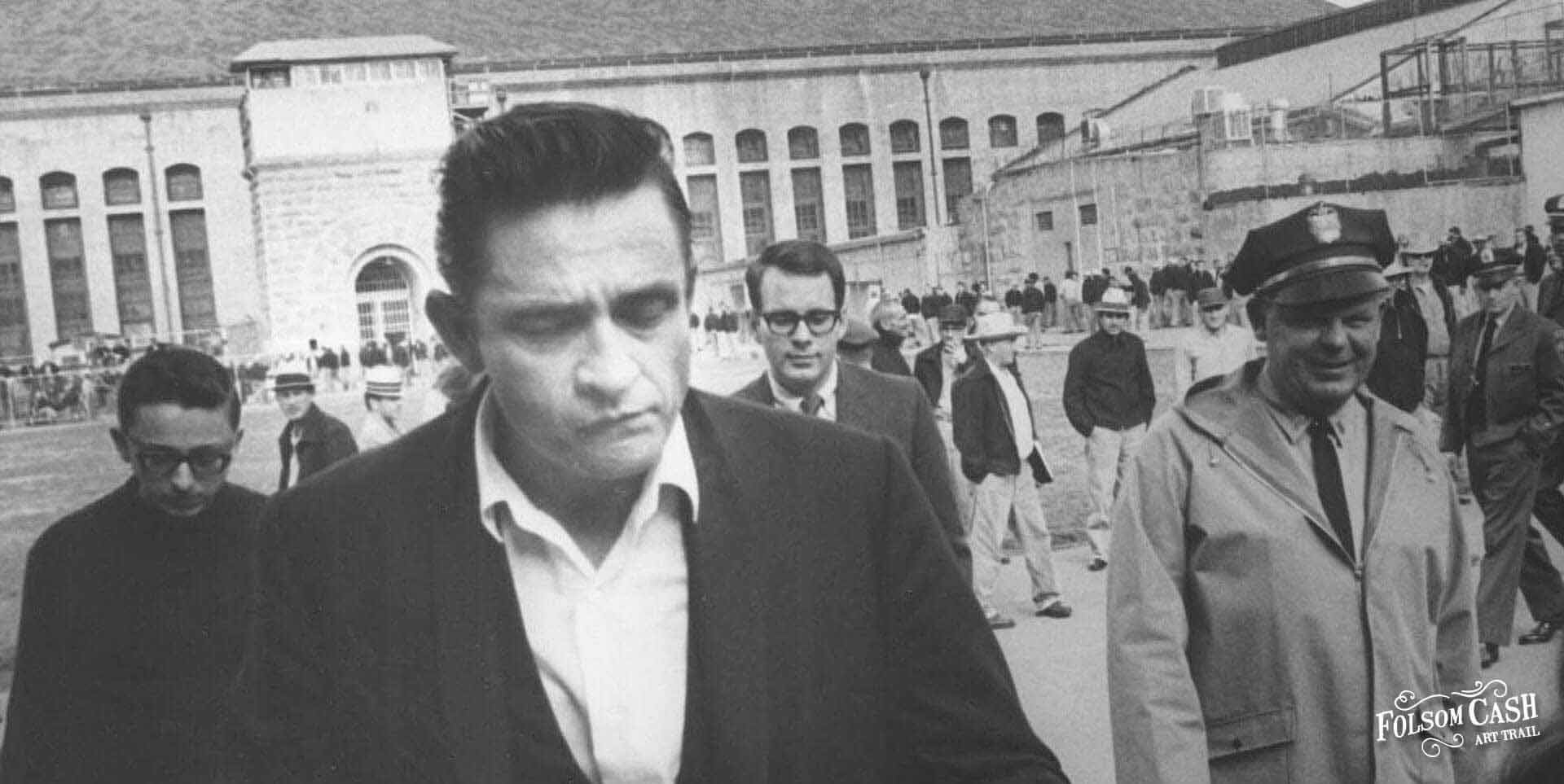This black-and-white photograph, likely from the 1960s or early 70s, vividly captures a significant moment, possibly at Folsom Prison. The central figure, reminiscent of Johnny Cash, stands out with his dark, slicked-back hair, closed eyes, and pursed lips. He wears a button-down white shirt and a dark jacket, exuding a timeless presence. In the background, numerous men are gathered, suggesting a bustling city square or the courtyard of a large institution, framed by expansive light-colored buildings or concrete and stone walls.

To his right and slightly behind, a police officer dressed in a traditional rain uniform coat with a distinctive old-fashioned hat observes the scene with a smirk. Another bespectacled man in a suit and several others form a dynamic backdrop, emphasizing the gravity of the moment. The ensemble of individuals, combined with the notable setting and the inscription "Folsom Cash" at the bottom, strongly hints at the historical event of Johnny Cash's legendary performance at Folsom Prison.